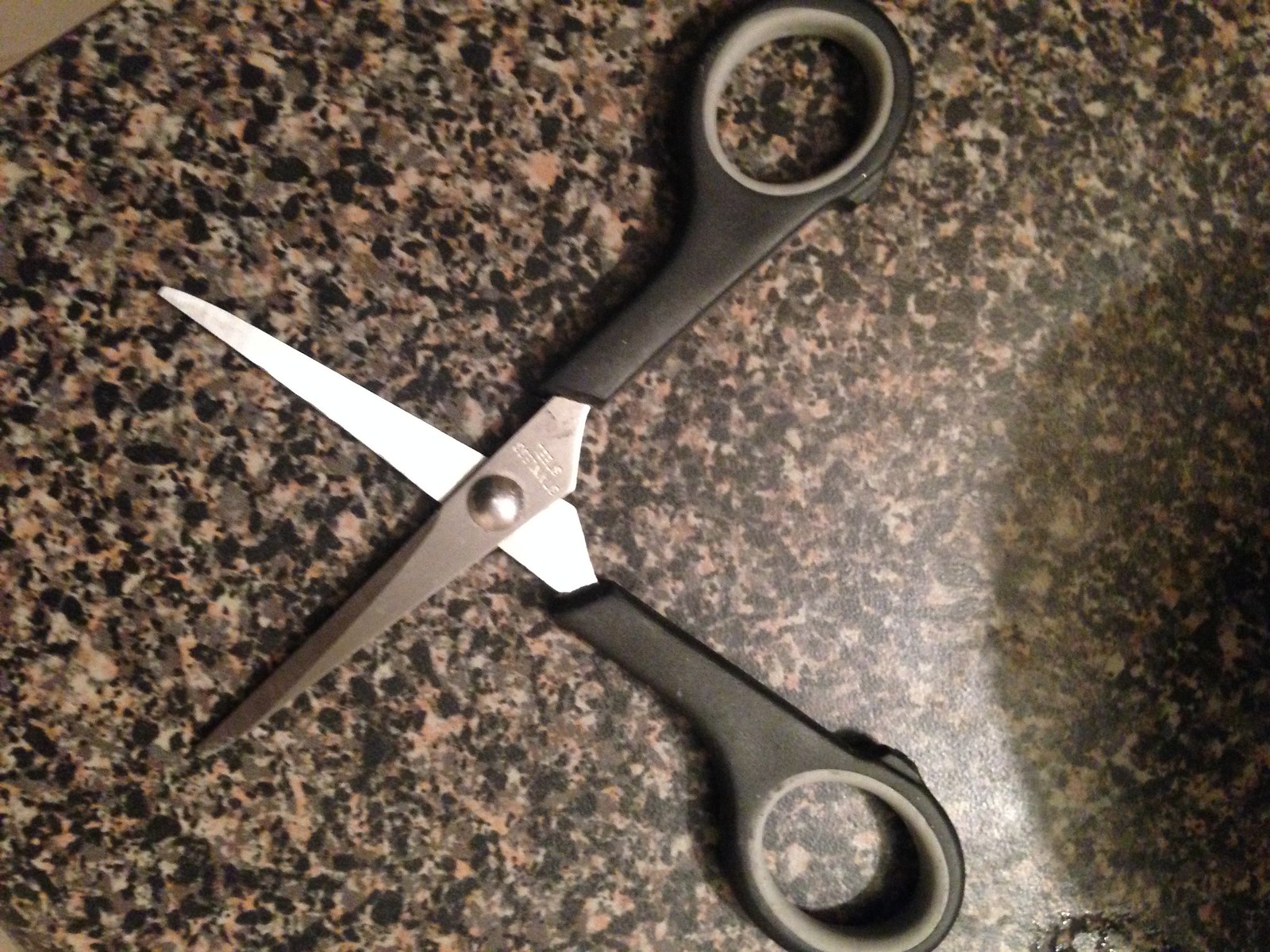This overhead photo features an open pair of scissors resting on a granite countertop with a mix of brown, white, gray, and predominantly black specks. The scissors, open with the blades facing left and handles to the right, have black handles with light gray inner comfort grips. The stainless steel blades are clean and relatively short, suitable for arts and crafts or child use. A shadow, likely cast by the person taking the photo, looms from the lower right corner. The edge of the countertop is visible in the upper right. The scene is well-lit, highlighting the detailed textures of the scissors and countertop, with no other objects present in the frame.